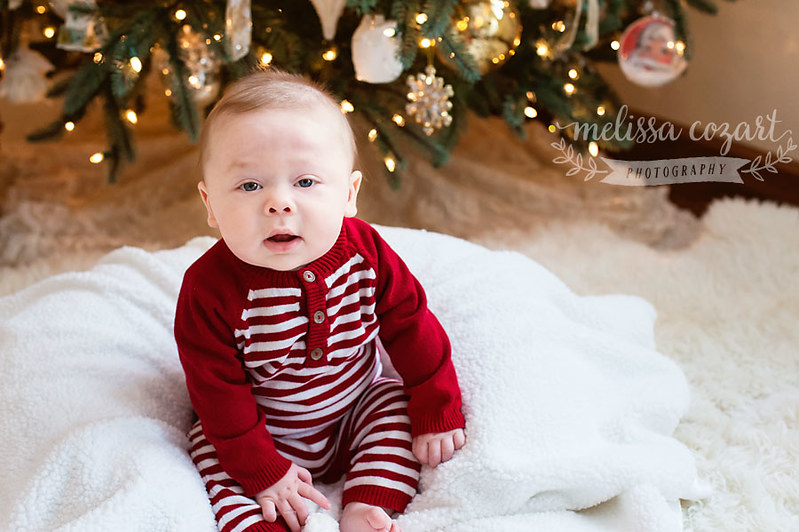A professionally taken photograph by Melissa Cozart Photography features a young baby, less than a year old, sitting on a white fluffy blanket or pillow. The baby is dressed in a festive red onesie with white stripes down the chest and front of the legs, complete with three buttons. His thin blond hair and blue eyes are prominently visible as he gazes sleepily at the camera. The baby is situated in front of a Christmas tree that's adorned with white lights, gold accents, and various ornaments including snowflakes and a Santa Claus face. The base of the tree is also surrounded by a white blanket, adding to the cozy holiday atmosphere. The photo includes a watermark in the upper right corner, reading "Melissa Cozart Photography" with decorative stems and leaves. The setting is softened additionally by a fluffy white carpet covering the floor.